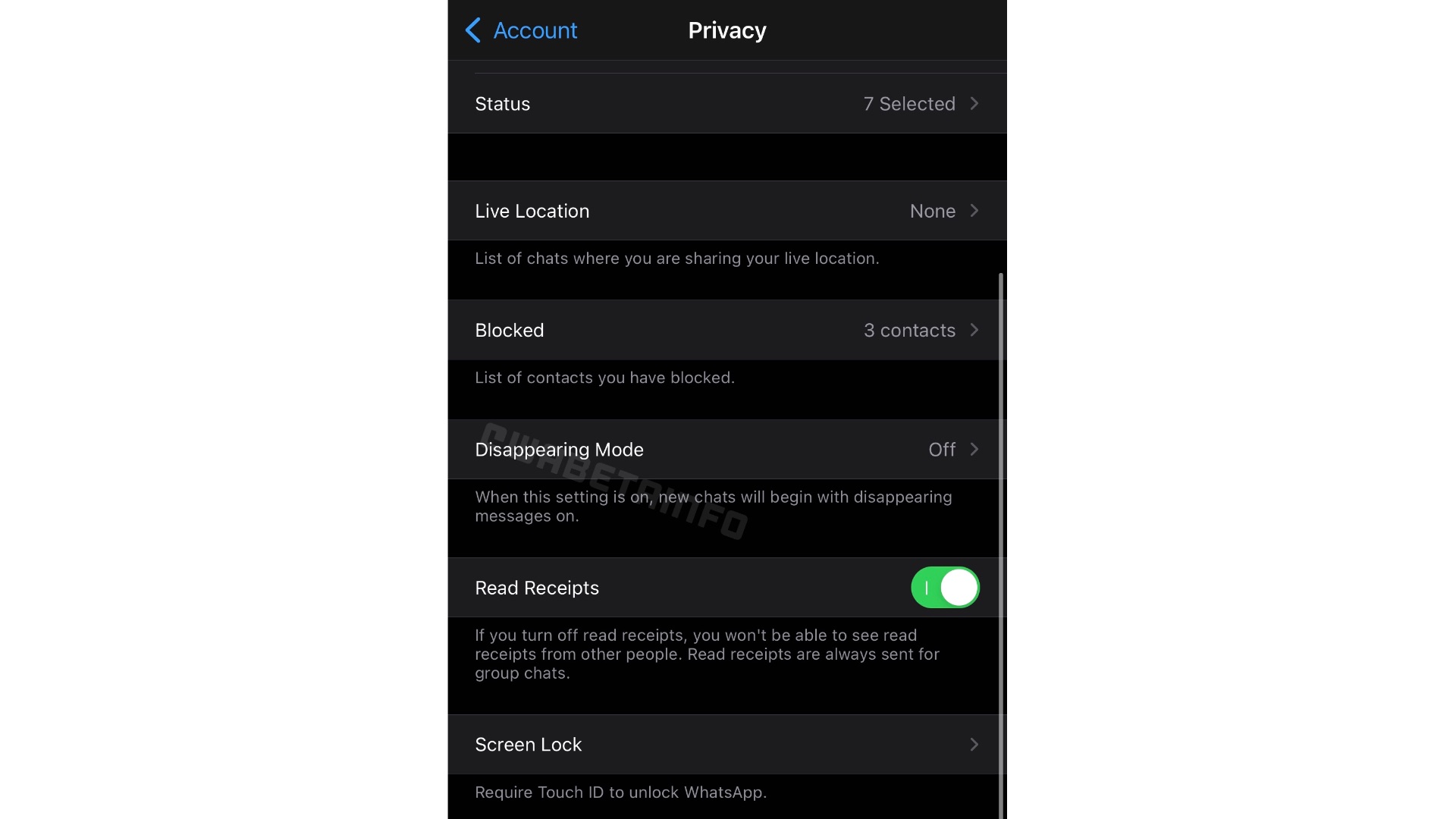Screenshot of a Privacy Settings Page

The image features a screenshot of a mobile application’s privacy settings page. The background is solid black, with blue and white text providing a clear and high-contrast visual. 

At the top, the word "Account" is displayed in blue font, accompanied by a back arrow. Below it, "Privacy" is written in white font. The page contains a series of black boxes with white text detailing different settings options.

1. **Status**: Displays "7 selected". This section likely allows the user to manage who can see their status updates.
2. **Live Location**: Indicates "List of chats where you are sharing your live location" with the status "None."
3. **Blocked**: Shows "List of contacts you have blocked" with the status "3 contacts are blocked."
4. **Disappearing Mode**: Explains that when this setting is on, new chats will begin with disappearing messages enabled. This feature is currently turned off. There is a pale gray watermark over this section.
5. **Read Receipts**: This setting is turned on (indicated by a green toggle with a white circle). It states, "If you turn off read receipts, you won’t be able to see read receipts from other people. Read receipts are always sent for group chats."
6. **Screen Lock**: Offers an option to require Touch ID to unlock the application, shown with a right-pointing arrow.

On the right side of the image, a gray scroll bar is visible, indicating the presence of additional settings that can be accessed by scrolling. The image quality is excellent—clear and sharp with no pixelation or blurring, ensuring all text and elements are easily readable. No other images or extraneous details are present.